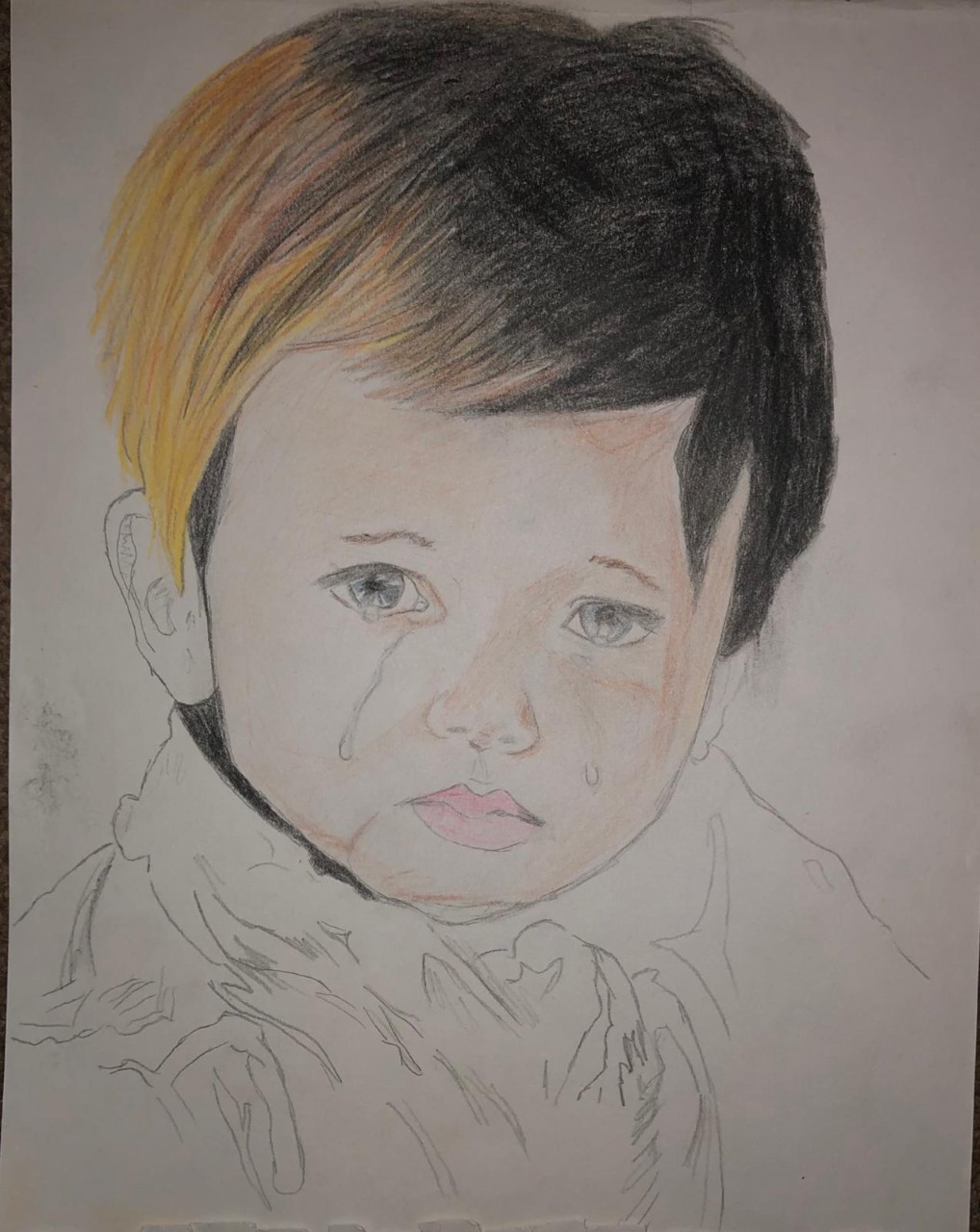This is a detailed drawing of a baby, likely a boy, showcasing a poignant expression. The child, who appears very young, has striking bluish-gray eyes filled with teardrops, mostly streaming from the left eye but with a few drops on the right as well. His slightly pink, full lips resemble those of a girl, adding to the ambiguity of the child's gender. Prominently visible is his left ear, with the right ear partially shown. His hair is a mix of brown and black, with a distinctive blonde highlight on the left side. The hairstyle is moderately short, neither too long nor too short.

The outfit the baby wears, depicted from the chest up, is sketched with pencil and left uncolored, contrasting with his subtly beige-white skin tone. The artist has detailed his facial features, including eyebrows and nose, which are easily discernible. His overall face shape is notably chubby, with a wider top tapering down to a slender bottom. This melancholic yet tender illustration vividly captures the innocence and delicate emotions of a young child.